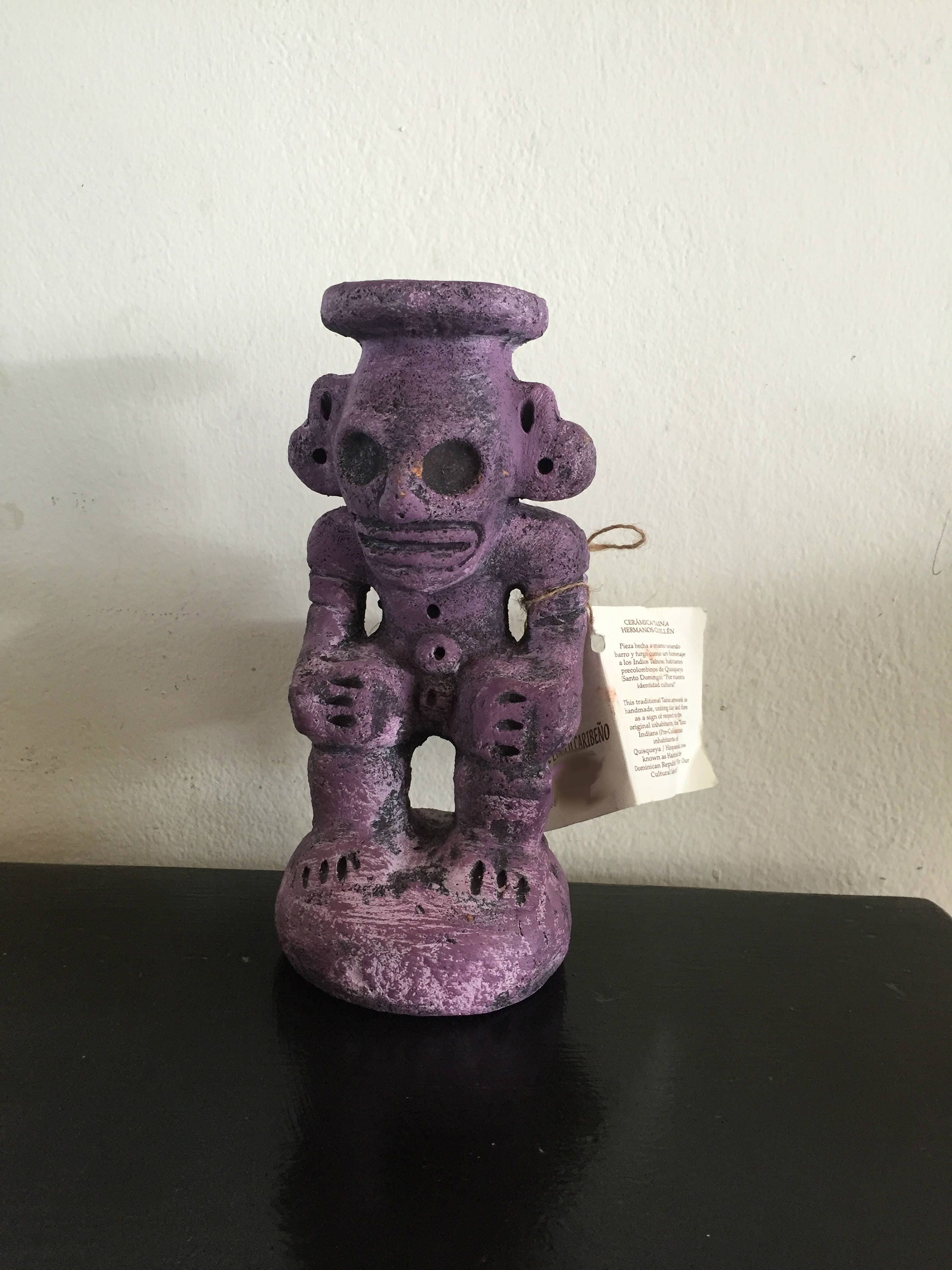The photograph captures a detailed image of an old, intricately carved statue set against a lightly textured eggshell white wall. Positioned slightly left of center on a dark-colored table, the statue portrays a humanoid figure in a squatting posture, with its wide feet, legs, and arms clearly defined. The figure's head merges into a vase-like disc, painted in a faded dark purple, revealing sections of the black material beneath due to wear and damage. The statue's facial features include a wide mouth with two simple, carved eyes, and it appears to be wearing a mask. Its midsection and ears are adorned with vertically aligned holes, enhancing its ancient and enigmatic appearance.

A noticeable detail is a paper tag attached to the left side of the statue, featuring black writing that is too small to read, possibly identifying the artifact. The left leg of the statue shows a slightly protruding knee, contributing to its lifelike squatting stance. The shadow of the statue is cast clearly on the left side of the photo, with a fainter shadow on the right, adding depth to the image.